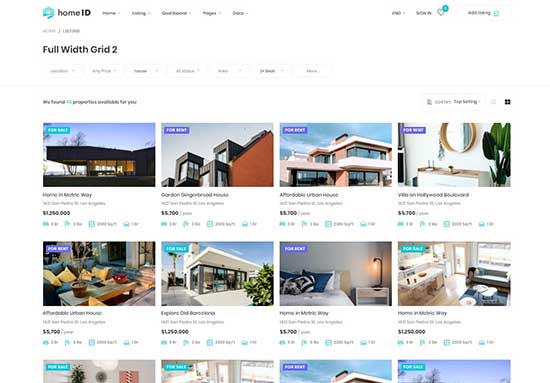This screenshot captures the homepage of a website named "Home ID." Prominently featured is a hexagonal blue logo depicting a sunset over a road. Adjacent to the logo is an extremely small, nearly illegible text menu presenting five options. In the upper right corner, there are elements for user sign-in and a heart icon indicating saved items count.

Below the main navigation, a section labeled "Full Width Grid Two" is visible alongside additional menu options. The primary content area displays listings for homes, organized into a grid with four columns and two fully visible rows, and a partially visible third row. Listings include both homes for sale and for rent, distinguished by colored buttons in the upper left corner of each image; teal for sale and purple for rent.

Each property image highlights key details such as exterior views and pricing. A home for sale is listed at $1.25 million, while a rental is priced at $5,700 per month. Beneath each image are various icons and text options, though the specific details are too small to discern. Overall, the site appears to facilitate rental and purchase transactions for residential properties.